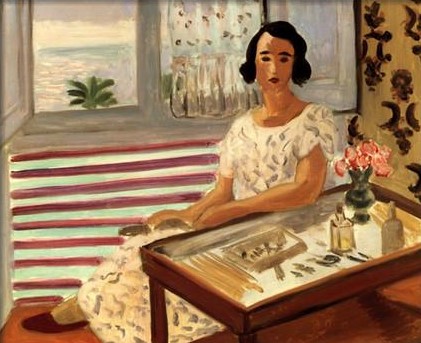The painting depicts a young woman with an olive skin tone and dark black hair, styled in buns on each side, seated in her living room. She is dressed in a white dress adorned with black music note shapes and is wearing red slip-on shoes. She is leaning her right arm on a glass top table while her left arm rests by her side. On the table, there are several items, including a clock device, a perfume box, a vase with red and slightly pink flowers that resemble roses, and an assortment of smaller objects such as a box of tissues and writing utensils. The window near her is open, revealing a view of the sea, a sky with palm trees, and eight pinkish floats in a pool. There is also a potted plant by the window. The setting includes a striped wall of blue and red and flowing white and red-gold curtains. The painting's style is uniquely balanced between realistic and simplistic, capturing a serene moment in a seemingly regular living room by the sea.